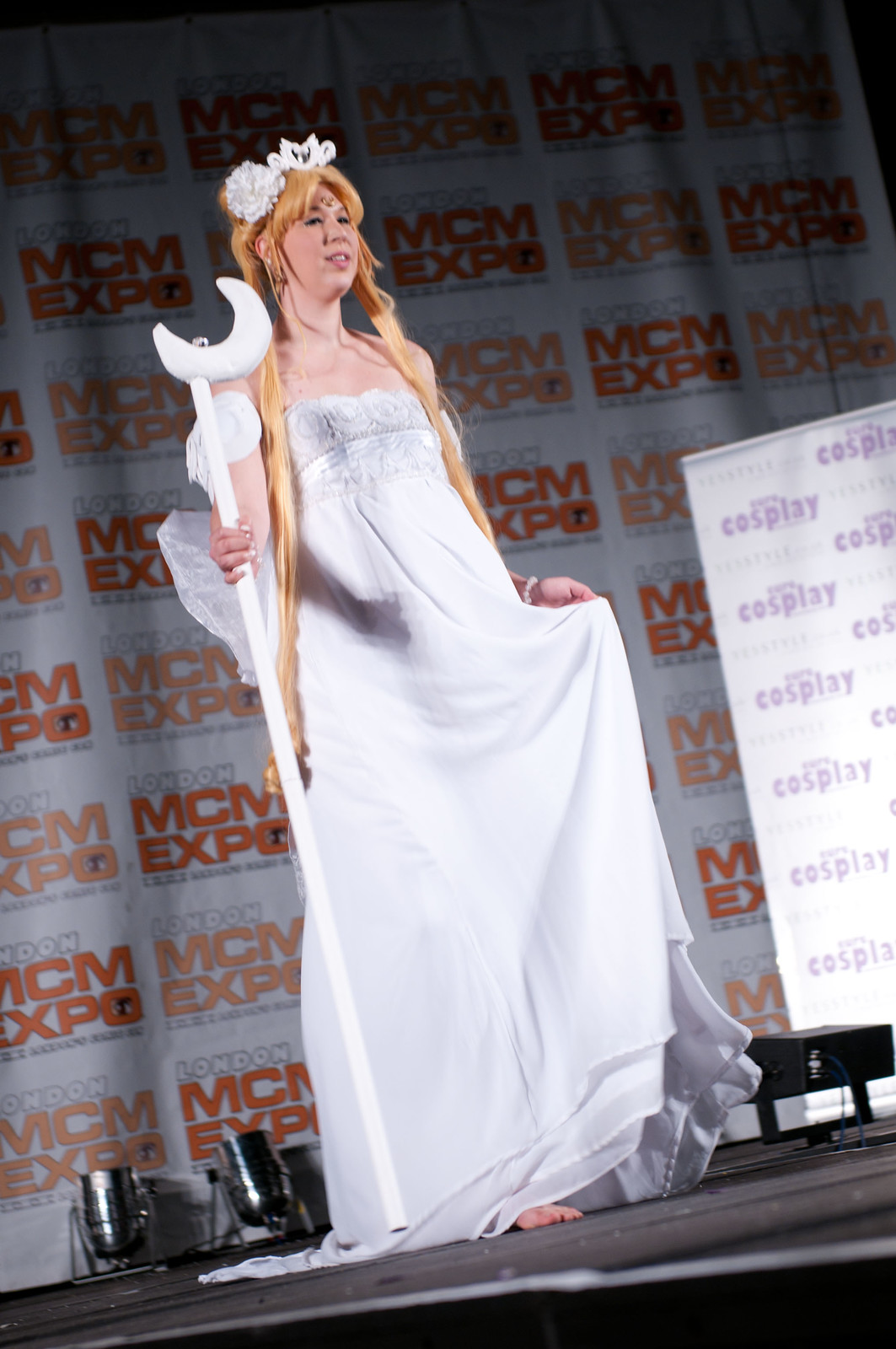The image depicts a woman on a stage at an MCM Expo event, as indicated by the orange MCM Expo logos that dominate the step and repeat background. She is dressed in a flowing white gown, reminiscent of a nightgown, and adorned with a white floral headdress. Her strikingly long, red hair, possibly a wig, cascades down her shoulders and over her hands. She is barefoot and holding a white staff topped with a crescent moon, suggesting she might be portraying a princess or mystical character in a cosplay competition. Additionally, there is a smaller step and repeat banner in purple reading "cosplay" multiple times. The stage floor is black, and there are silver spotlights directed upwards. There's also a black projector on the floor, adding to the technical setup of the event. Overall, the detailed attire and the themed background strongly indicate that she is participating in an official cosplay convention.